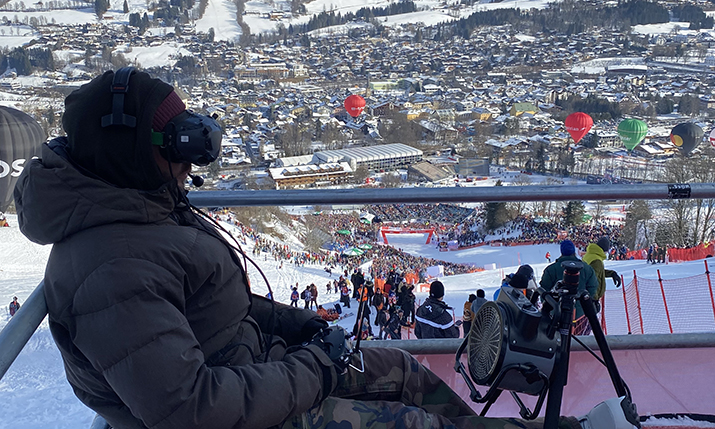The image captures a bustling ski resort scene from an elevated perspective, offering a panoramic view of the snowy landscape below. Dominating the foreground is a person dressed in a gray puffy coat with a black hoodie and a red beanie. This individual, possibly a broadcaster or a skier, is wearing a headset with a microphone and holds a controller, suggesting she might be engaging in some sort of commentary or virtual skiing experience. Adjacent to her is a fan or heater, perhaps to keep her warm in the wintry conditions. Her attire also includes camouflage-patterned pants in shades of green and brown.

In the background, a multitude of people scattered across the snowy terrain appear tiny, akin to ants from this vantage point. The scene includes a vividly colored collection of hot-air balloons—a couple red, one green, and one black, with another balloon in the leftmost part of the image possibly featuring a MasterCard logo with red and yellow circles.

The setting appears enveloped in a scenic, snow-covered city, dotted with numerous houses and tents, adding to the picturesque and eventful atmosphere.